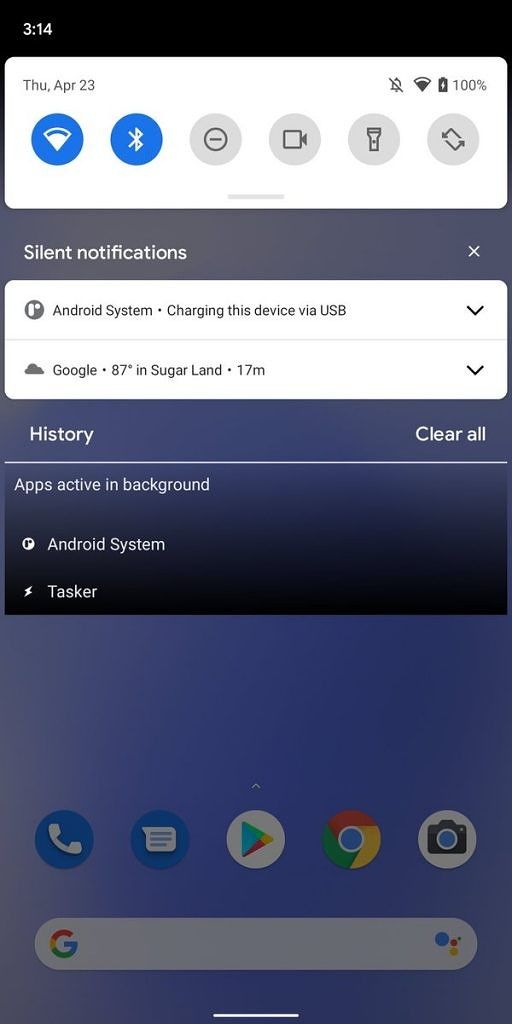A mobile phone screen displaying several silent notifications appears to be the focal point of the image. The device is an Android system, currently being charged via USB. The weather widget shows a temperature of 87 degrees in Sugar Land. A "history" button is visible, along with an option to clear all notifications. Multiple apps are active in the background, including the Android system and Tasker, though their specific activities are not clear. Standard navigation buttons are present at the bottom of the screen, such as "Make a Call," an unidentified icon, the Play Store, Google, and the Camera, none of which are currently highlighted. The Google search bar is also present but not highlighted. Notably, the only illuminated item is an "Android Aura" notification, indicating that the device is charging. It seems the primary activity being performed is charging the phone.